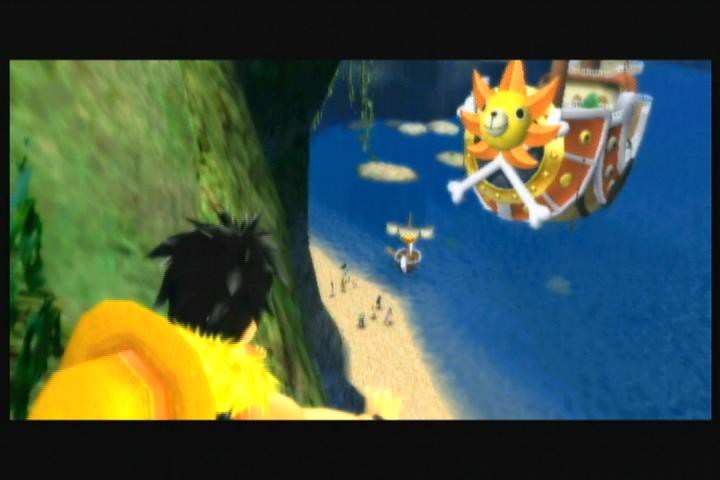The image is a detailed screenshot from what appears to be either a video game or an animated show, likely "One Piece." The main focus is on a large pirate ship prominently featuring a giant teddy bear-like sun on its bow. The pirate ship is primarily dark brown with accents of tan and green towards the rear. The teddy bear sun, encircled by a gold outline and set against a dark blue background, boasts a black nose with a beige tip, a mouth lined vertically and horizontally, and two large, beady black eyes. Its rays are stylized as curved orange triangles, giving it a vibrant appearance. Beneath the sun, two crossed bones are visible. To the left, smaller tan-colored ships, blurred due to distance, anchor near a sandy beach. The water surrounding them is dark blue, dotted with small tan islands, and bordered by dark green plant foliage and a grayish cliff edge.

In the foreground, an individual with short black hair and a frilly yellow shirt is visible from behind. A wicker hat adorned with a red ribbon rests on their back. This character appears to be observing the scene, adding a human element to the otherwise nautical setting. Surrounding the scene are green trees, grass, and other island elements, creating a rich and dynamic composition.